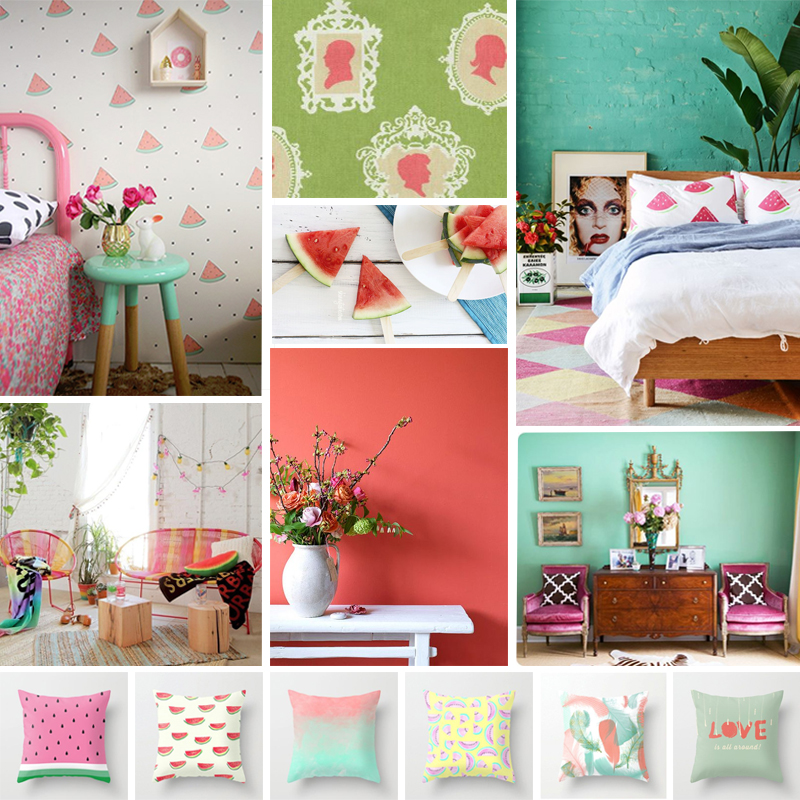The image is a detailed collage of home decor visuals emphasizing a watermelon theme across nine panels. In the top left corner, three images in a vertical column showcase a bedroom adorned with watermelon wallpaper and a pink bed, followed by a living room with watermelon-colored furniture including a noticeable watermelon pillow, and lastly, two distinct watermelon-themed pillows, one resembling the inside of a watermelon with a green stripe and the other featuring small watermelon patterns.

In the middle column, from top to bottom, a green wall with classic pink silhouettes is displayed, followed by a stylish layout of watermelon slices on popsicle sticks, and further down, a watermelon-colored wall contrasted with a white table holding a bouquet of flowers in a white pot.

The right column reveals a bedroom with pillows depicting watermelon slices, a room furnished with pink chairs and green watermelon-themed wall decor, and the lowest image in this column is somewhat indistinct but appears to contain more accent pillows.

Finally, a strip of six smaller squares at the bottom shows various pillow designs, including two with watermelon patterns, a red and blue gradient design, a yellow field with rainbow motifs, an abstract paint-like design on a white background, and a green pillow emblazoned with the word “LOVE.” This thoughtful arrangement allows for a comprehensive view of how the watermelon theme and coordinating decor elements can be harmoniously integrated into different living spaces.